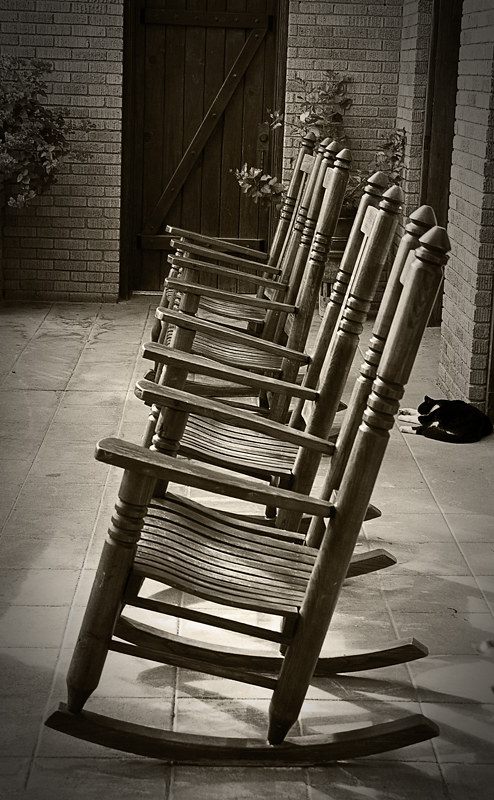This image captures a line of four wooden rocking chairs, artistically composed on an outdoor patio paved with square pavers. The chairs, painted a weathered gray, are positioned in a straight row, facing left. They feature slatted seats and backs, and intricate wood carvings on the sides. The setting includes walls of rustic gray brick on the back and right, adding texture to the scene. A diagonal-braced wooden door is visibly attractive against the back wall, enhancing the rustic charm. In the corner, a potted tree adds a touch of greenery, while another house plant peeks into the frame from the upper left-hand corner. A black cat with white markings and paws is curled up asleep against the right wall, contributing a relaxed, homely feel to the composition.